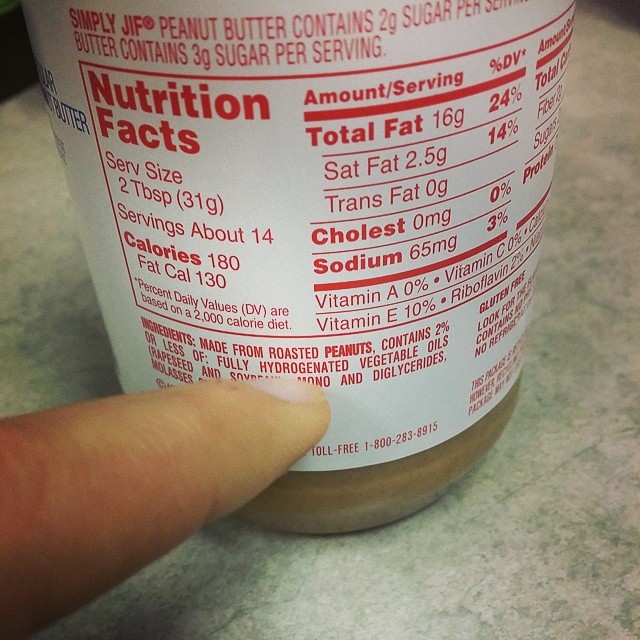In this detailed photograph, a person's left hand is prominently pointing to the ingredient list on the Nutrition Facts label of a Simply Jif peanut butter container. The index finger is specifically highlighting the word "hydrogenated," which appears as part of "hydrogenated vegetable oils" in the list of ingredients. The label prominently displays various nutritional details, including a serving size of two tablespoons, alongside information on calories, fat, cholesterol, sodium, and other typical nutritional breakdowns. The container is made of plastic, and though the image primarily focuses on the label, the peanut butter product is faintly visible below the label at the bottom of the photo; however, the top part of the container, including the lid, is not visible in the frame. The scene is set against a green and white countertop, adding a contextual background that contrasts with the packaging.